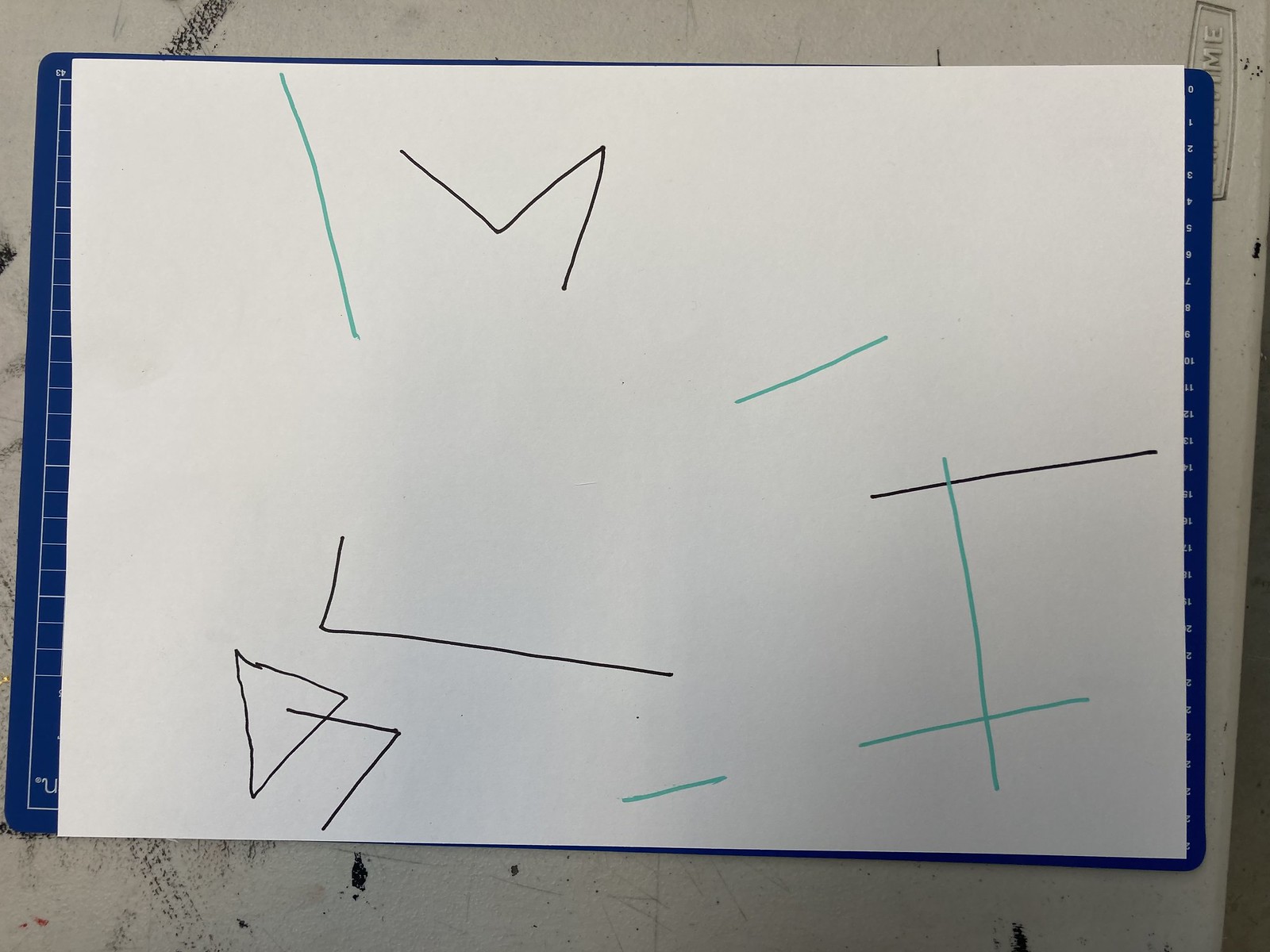The image features a blank piece of white paper placed on a blue grid background. The paper is adorned with various black and green sketches, primarily consisting of lines and rudimentary shapes. In the top section, a green diagonal line tilts to the left, accompanied by a black zigzag line. The bottom portion of the paper showcases a black triangle, with an unfinished black triangle missing one side positioned above it. Additionally, the bottom right corner of the paper features a sketch of an eye, predominantly in green, but with a black horizontal line across the top. The white countertop beneath the paper exhibits some scratches. The overall arrangement on the paper includes both long and short lines, creating a mix of detailed and simple elements.